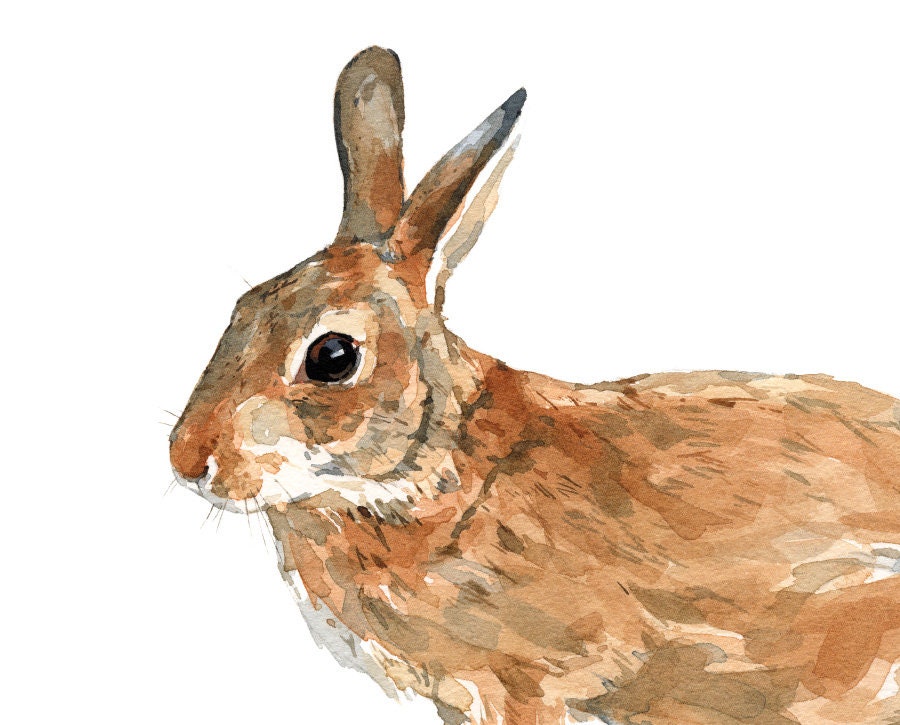This is a beautifully detailed watercolor painting of a hare against an entirely white background. The painting appears to be done over a subtly textured white canvas. The hare, primarily adorned with brown and gray fur, is depicted facing the left side, with its large ears perked up above its head, showcasing gray and brown exteriors and white interiors. Only one dark, almost black eye is visible, detailed with hints of brown. The hare's nose is brown, and the area around its mouth and chin is white. Unique to the hare are its twelve whiskers, standing out against the detailed fur. The body extends to the right, displaying a variety of brown shades with subtle hints of olive gray, becoming less detailed and more impressionistic as it reaches the edge of the canvas. The strokes of the paint are visible, adding texture, and the right side of the hare is cut off, suggesting it continues beyond the boundary of the image, creating a dynamic and engaging composition.